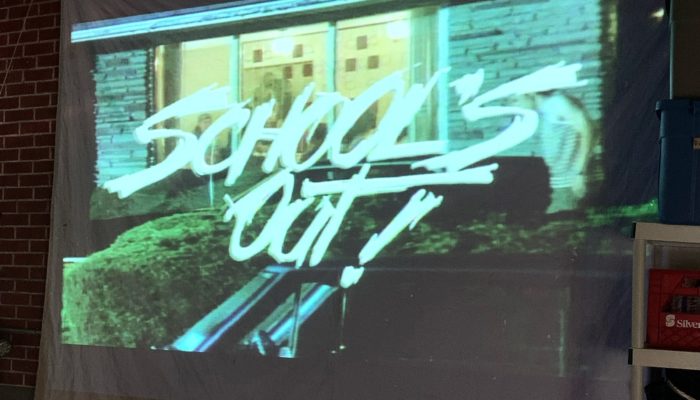The photograph captures a projected image on a fabric screen pulled down in a classroom, anchored onto a brick wall in the background. The projection showcases a low-definition exterior scene of a vintage 70s brick house, partially illuminated by what could be moonlight, with the brickwork giving off a silvery-gray hue. Dominating the image is the bold, haphazardly written text "Schools Out!", possibly referring to a celebration or an announcement. Below this text is the top portion of a black car, with neatly manicured green shrubs situated between the vehicle and the house. The house features a large, three-pane golden window, revealing art pieces on the interior walls and faint figures inside. On the right side of the projection, a blurred figure walks past the house. Surrounding the screen within the classroom, the exposed brick wall is visible on the left, while the right side has a small white shelf holding a red box and a black storage tote.